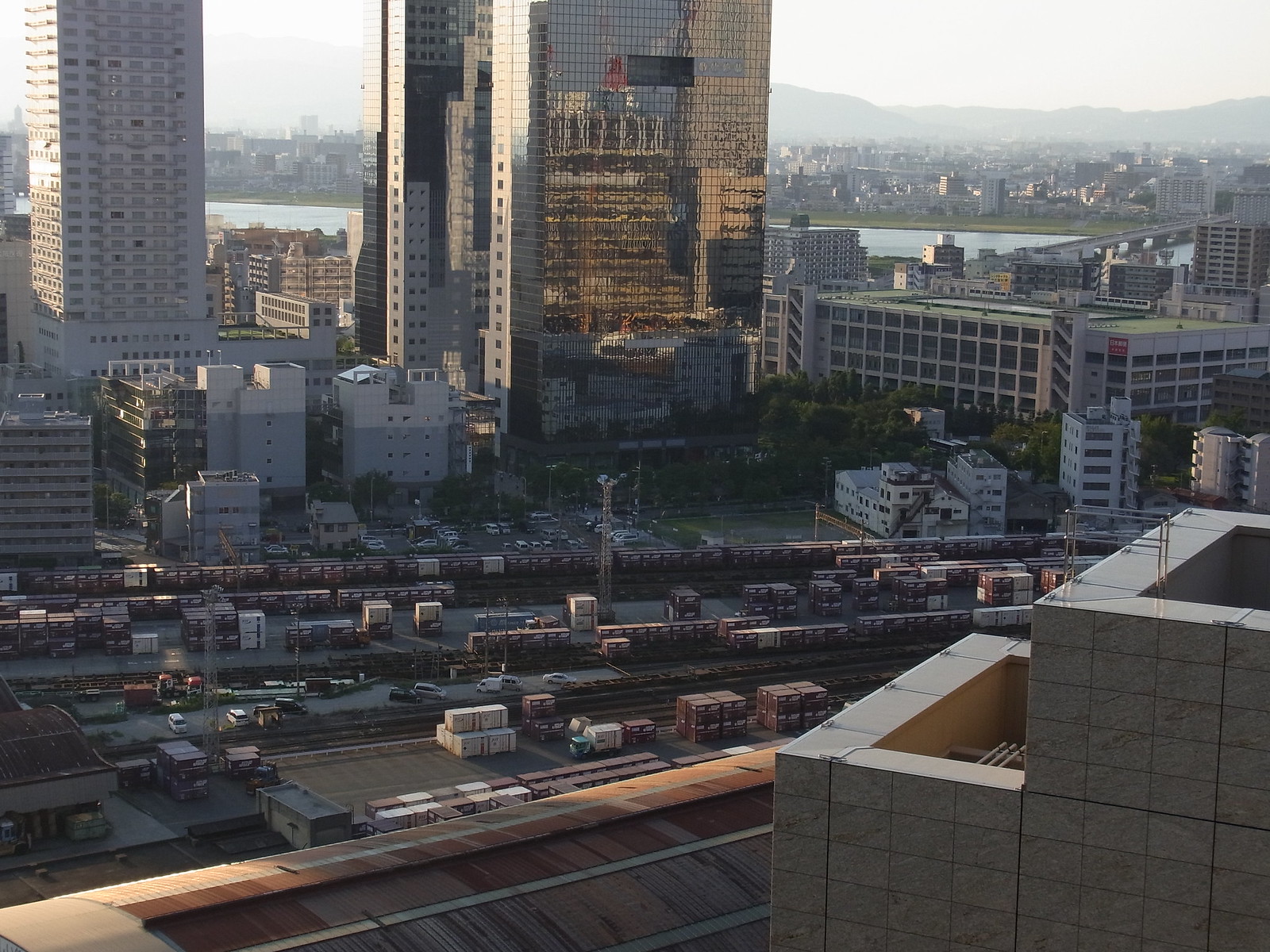The image captures a high vantage view of a bustling cityscape. Centrally positioned is a sprawling storage yard crowded with numerous shipping containers, train carriages, construction supplies, and stacks of cargo, giving an impression of a busy industrial hub. Tiny trucks are barely discernible amid the vast assortment of materials. In the bottom right corner stands a gray stone building with visible upper levels, and a rusted metal roof runs along the lower edge of the image. The storage yard is flanked by several towering structures, including a prominent skyscraper adorned with reflective windows that shimmer with silver and copper hues. To the left of this skyscraper is another high-rise with a distinct white facade. In the distance, a river snakes from the upper left to the upper right of the image, bordered by additional large buildings on both banks. Far into the horizon, a series of mountains and hills rise, creating a scenic backdrop to the expansive urban landscape.